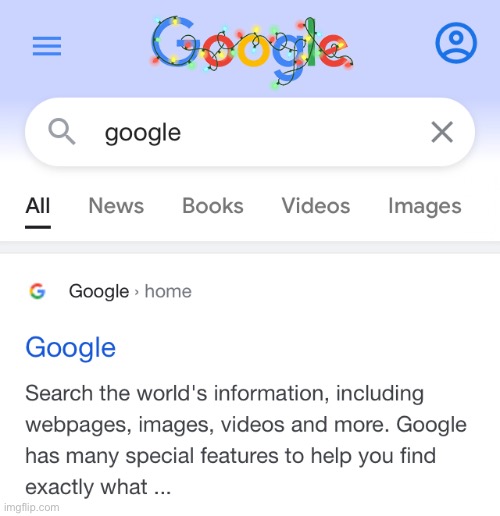The image depicts a Google search homepage decorated for Christmas. The iconic Google logo at the top is adorned with festive Christmas lights, suggesting it was displayed during the holiday season. 

To the left of the logo, there are three blue dashed lines, likely representing a menu icon. On the right side, there is a circular user icon. Below the logo, "Google" appears within a text box, with a magnifying glass icon on the left indicating a search function, and an 'X' icon on the right, probably for clearing the search box.

Directly beneath the search bar are navigation buttons labeled "All," "News," "Books," "Videos," and "Images." Further down, the word "Google" is again visible alongside "Home." Below this, there is text in blue reading "Google," followed by a description that says, "Search the world's information, including webpages, images, videos, and more. Google has many special features to help you find exactly what..." indicating a cut-off preview of information describing Google's search capabilities. 

The overall layout of the page features a predominantly white background, with the upper section in blue and the text in black or gray. At the bottom left corner, there is a watermark from "imgflip.com."

This summary captures a festive, user-friendly Google search homepage with both holiday spirit and functional design.